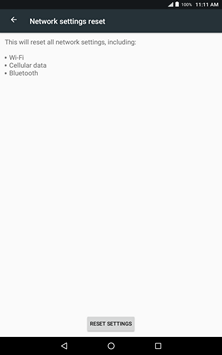In this somewhat blurry smartphone screenshot, the time displayed in the top-right corner reads 11:11 a.m., accompanied by icons indicating full network strength and battery life at 100%. These icons are white against a black background. Below this status bar, the phone shows a screen related to network settings reset, with a dark blue header highlighting the title "Network settings reset" in white text.

The main part of the screen displays a light gray background with black text, explaining, "This will reset all network settings, including Wi-Fi, cellular data, Bluetooth." At the bottom of this section is a gray button with "Reset settings" written in black, indicating the user can press it to proceed with the reset.

At the very bottom of the screen, the standard smartphone navigation buttons are visible against a black background: a left-facing triangle for "Back," a circle for "Home," and a square for "Overview" or "Recent Apps." The entire screen is centered around the functionality of resetting network settings, making it clear that pressing the "Reset settings" button will initiate the process, affecting Wi-Fi, cellular data, and Bluetooth configurations.